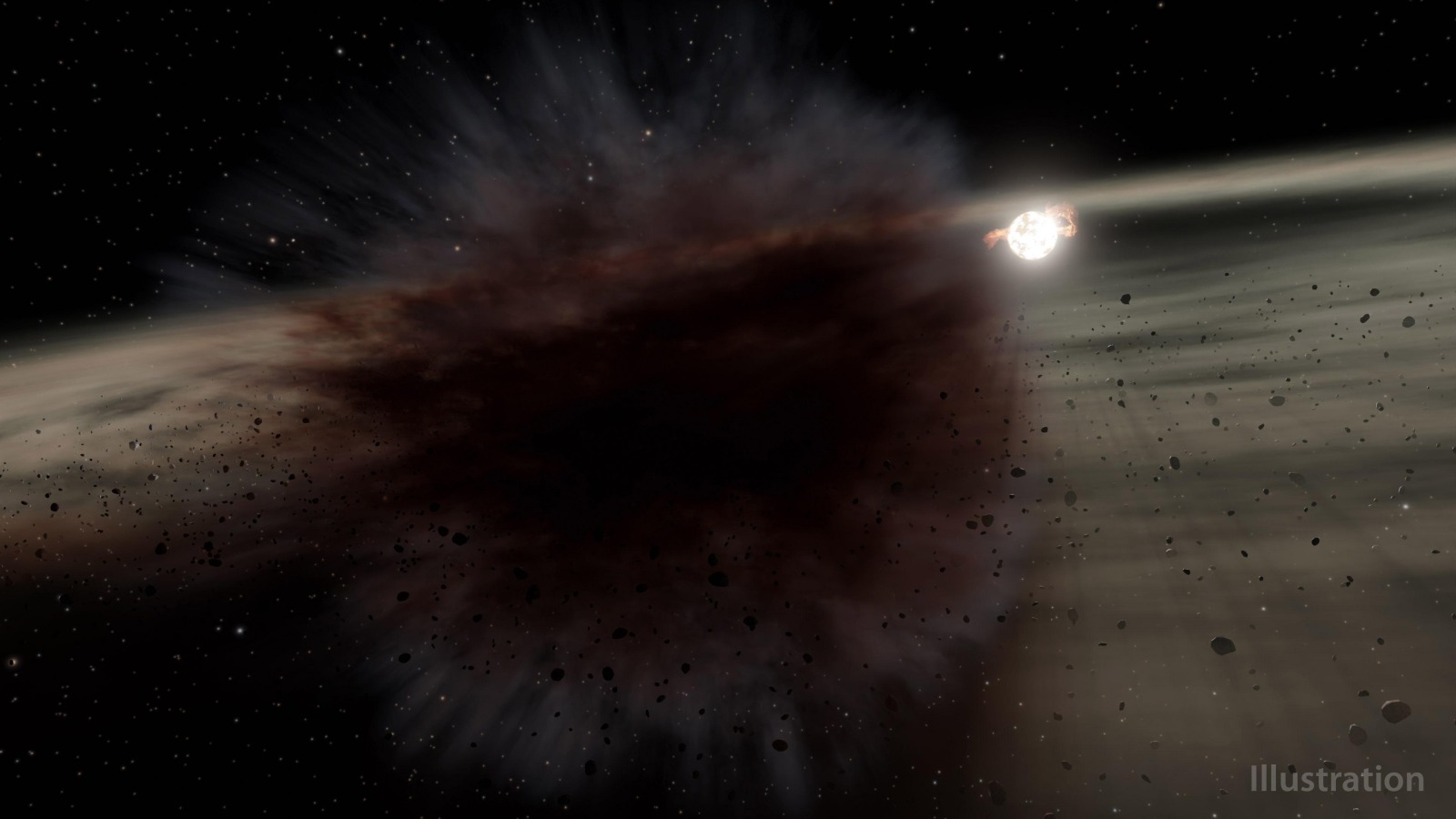The image portrays a detailed pixel art illustration of an astronomical event viewed from orbit. Dominating the lower half is the horizon of a grayish planet, showcasing its curvature and a textured surface with darker gray cross-hatching. At the horizon's edge, a small, bright white moon or planetoid is visible. Above the planet, the blackness of outer space stretches outward, punctuated by a sparse scattering of white stars. 

In the upper half, the centerpiece is a dramatic, deep burgundy red explosion, almost bloody in hue, with wispy white lines radiating from its circular form, consuming a portion of the sky. The explosion is surrounded by numerous small stone fragments, seemingly propelled outward from the blast. Adjacent to this scene on the right, a glowing white orb contrasts sharply against the dark background, appearing small yet intensely luminous.

Subtle details include a brown, cloudy area near the explosion that adds to the depth and complexity of the scene. In the lower right corner, the word "illustration" is inscribed in grayish white text, affirming the artwork's imaginative nature. The overall composition is dark, evocative of a nighttime scene in outer space, capturing both the serene and violent phenomena of the cosmos.